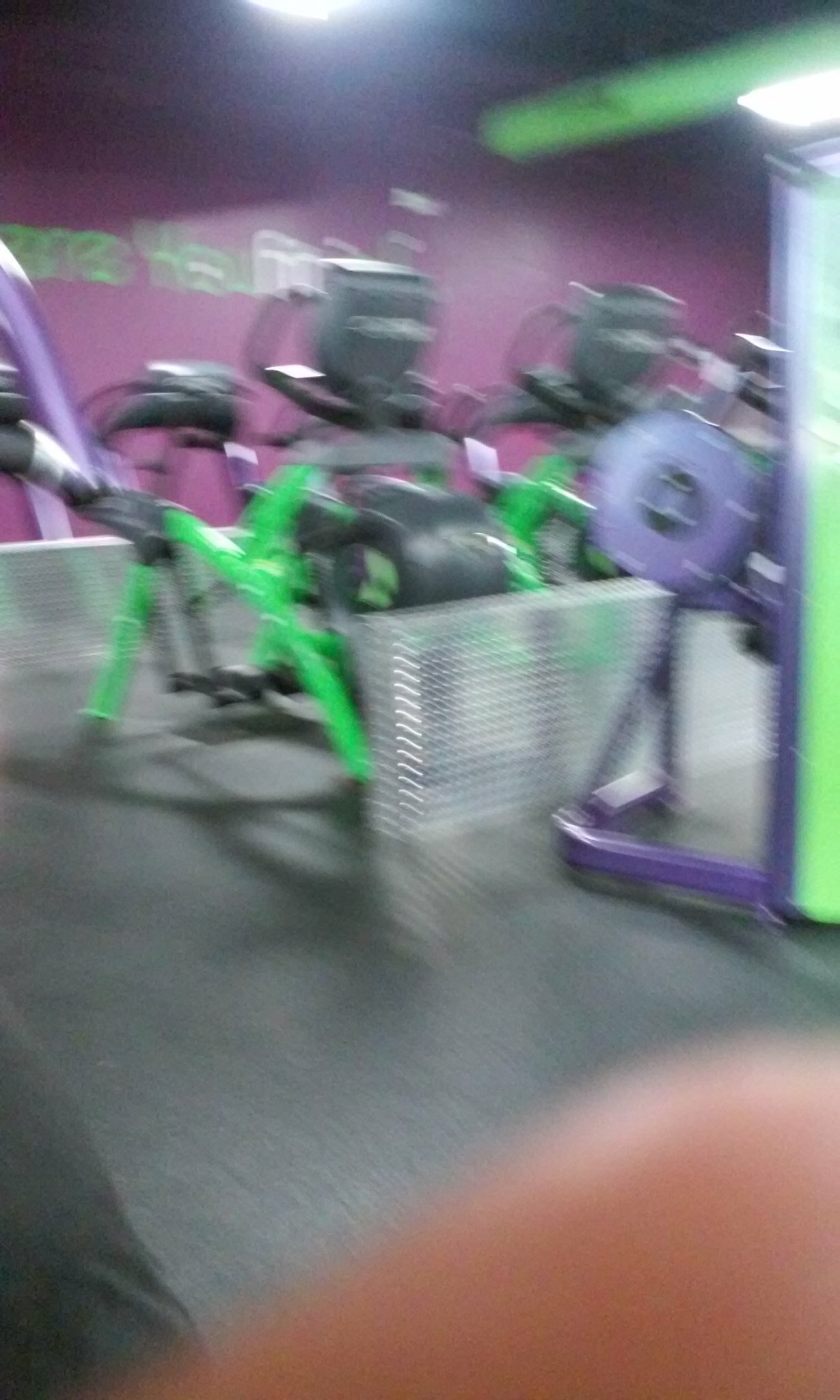This color photograph is significantly out of focus, creating a very fuzzy and blurry image that suggests the camera was shaking when it was taken. The scene appears to be the interior of a gym or workout area, identifiable primarily by its distinctive elements. The wall is painted a vibrant purple, and though there is some green text on it, the text is illegible. The floor is black, which contrasts with what seems to be workout equipment or machinery, primarily in black, purple, and lime green hues. At the center of the image, there's a large silver box that has a corrugated, automotive chrome-like appearance. Additionally, at the very bottom of the photograph, there is a flesh-colored indistinct blob, which could possibly be a finger or knee, but it is difficult to determine due to the lack of clarity.